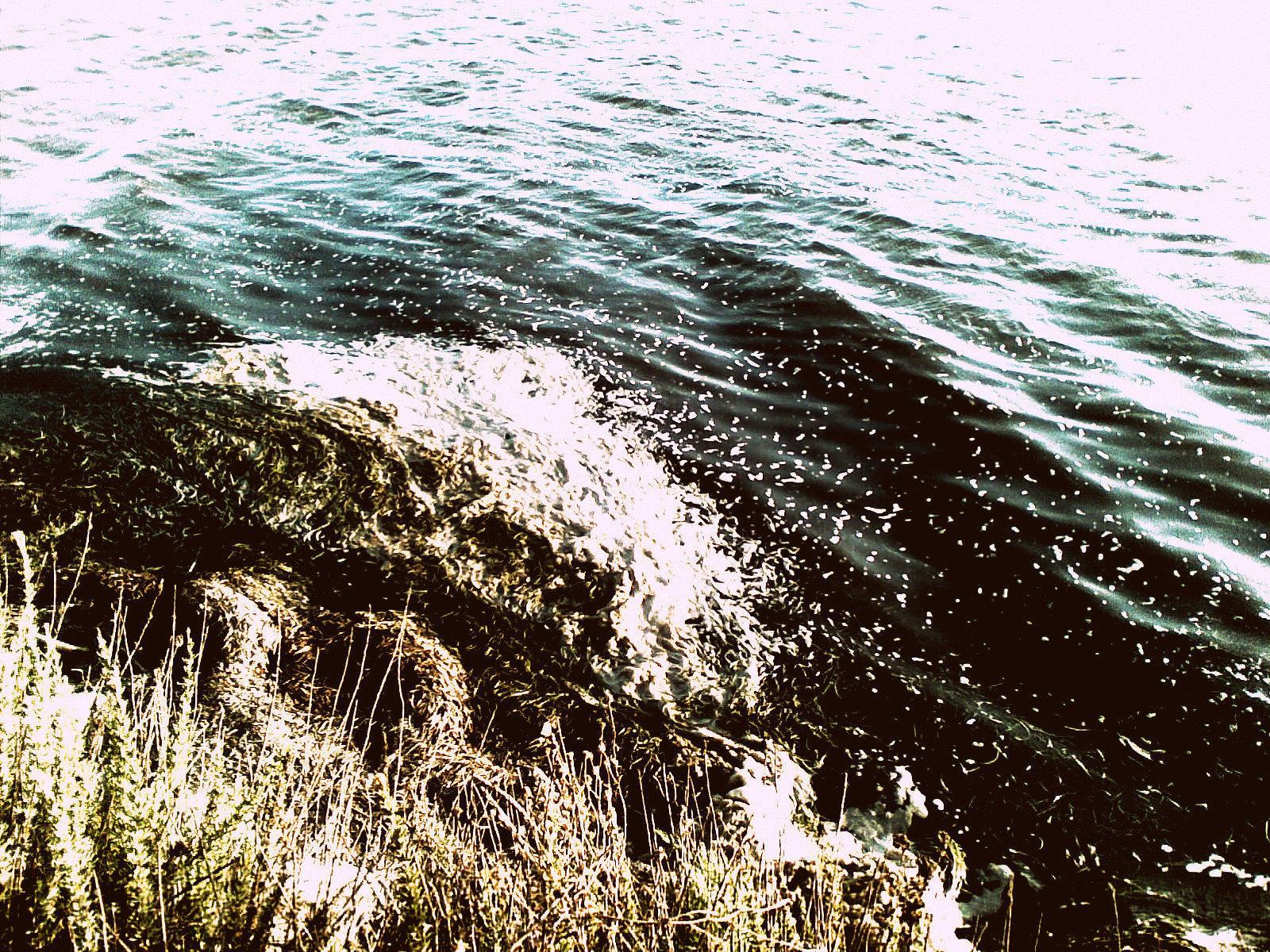In this vivid and detailed outdoor scene, the central focus is on water crashing against a large rocky shoreline to the left. The rocks, primarily a wet, watery brown, glisten as the water splashes against them, transitioning to a darker, almost black hue when catching the sunlight. Soft waves gently roll towards these rocks from the center-right, creating a slight foamy appearance among the ripples of the dark greenish water. Closer to the viewer, a cluster of dried, white weeds and plant life, interspersed with light green and brown leaves, emerges from the water’s edge, giving the scene a sense of natural, untamed beauty. In the background, the water changes color, shifting from its darker tones to a lighter purplish-white where the sunlight touches it, suggesting a serene, calm atmosphere. This picturesque shoreline, captured likely at midday, might be part of a lake, river, or coastal area, with the sunlight enhancing the vivid contrasts and textures of the rocks, water, and vegetation.